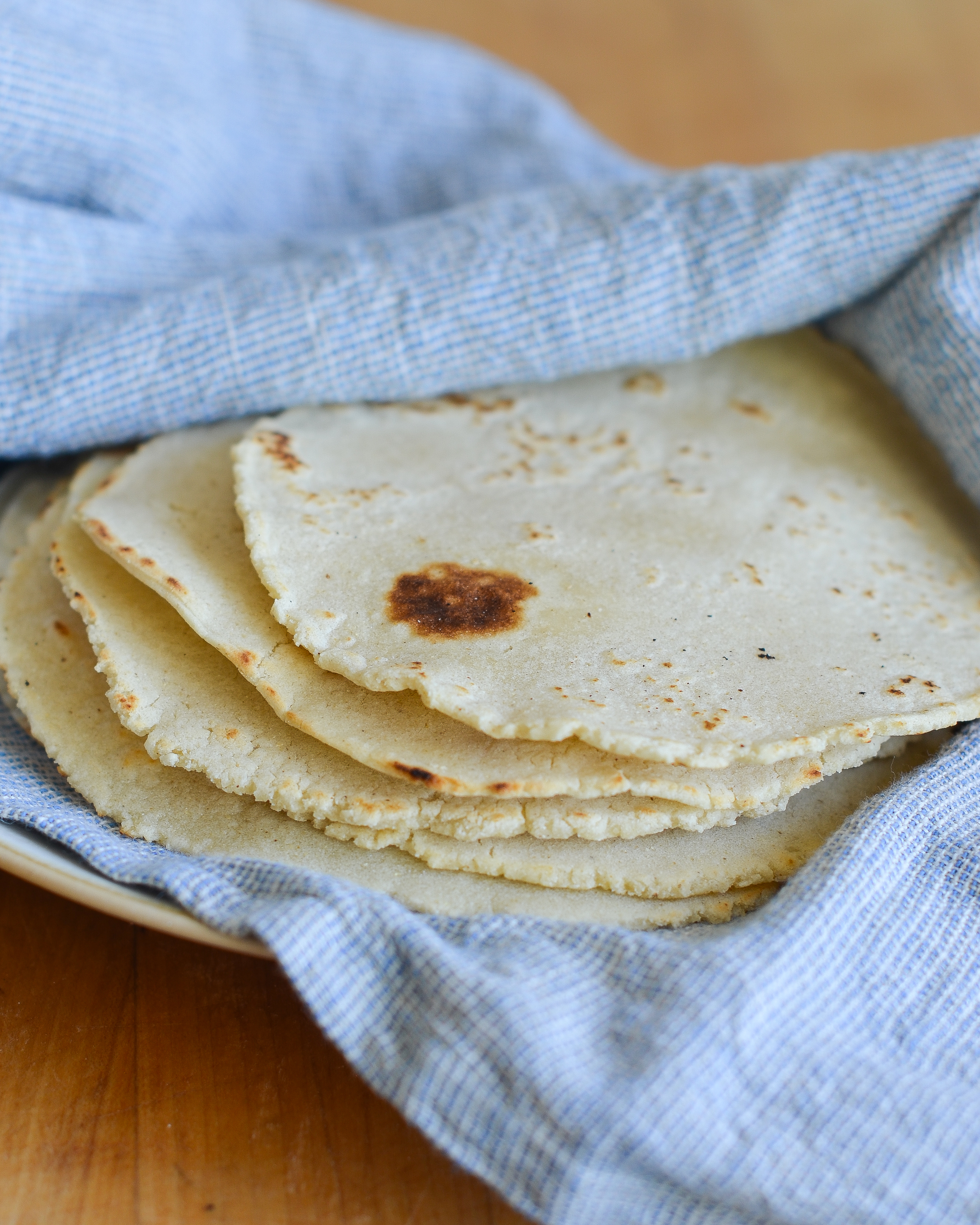This photograph depicts a stack of five medium-sized homemade flour tortillas partially wrapped in a light blue, thin but sturdy cloth, resting on a cream-colored plate. The tortillas display the characteristic brown spots from cooking in a frying pan, with the top one showcasing a particularly large brown mark on its left side. Additionally, small charcoal pieces, about three millimeters thick, are scattered atop the tortillas. The scene is set indoors against a light brown wooden table, emphasizing a cozy and inviting atmosphere perfect for enjoying these delicious, freshly made tortillas.